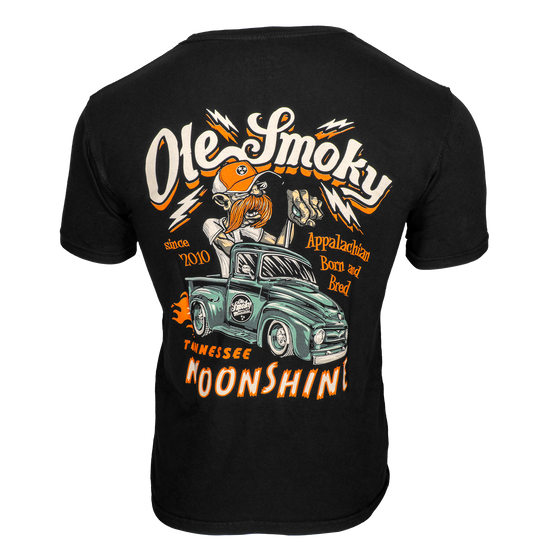This detailed color photograph captures the back of a black short-sleeved t-shirt set against a white background. The top of the t-shirt features the words "Ole Smokey" written in elegant white script, surrounded by four white lightning bolts. Beneath it, a similar "shadow" design is repeated in yellow. Dominating the center of the shirt is a vibrant illustration of a man with a large bushy orange mustache, wearing glasses and an orange and white baseball cap adorned with three stars inside a black circle, which is the state logo for Tennessee. The man, clad in a short-sleeved white shirt, is driving a distinctive green pickup truck with a flatbed, equipped with protective sides and a conspicuous gear shift protruding from the roof. Orange flames burst from the back of the truck, adding a dynamic flair. Flanking the illustration are notable text elements in orange and white: to the left, "Since 2010;" to the right, "Appalachian Born and Bred." Below the truck, "Tennessee" is written in orange text, while "Moonshine" follows in white.